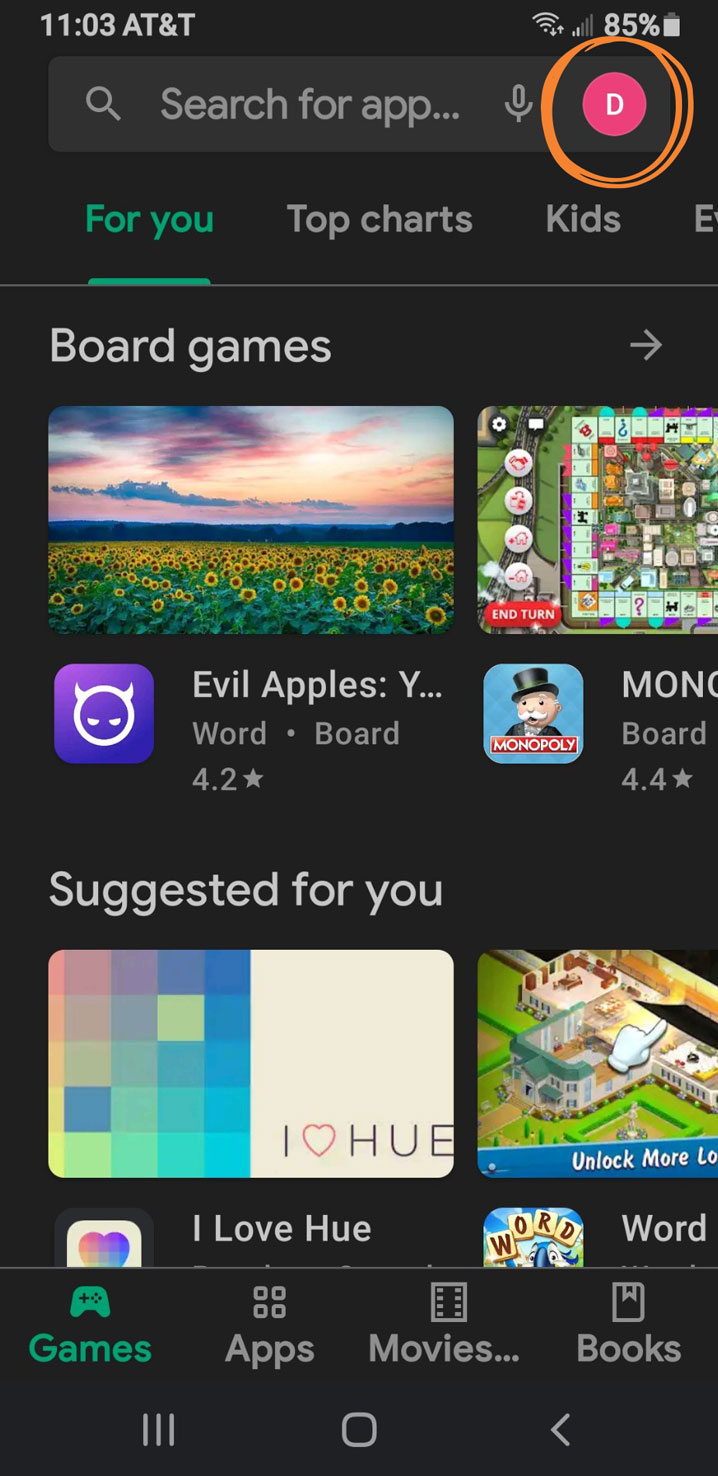A smartphone screen displaying various features and categories of a digital storefront. The time at the top of the screen shows 11:03, and the mobile network service is AT&T with a battery level of 85%. At the top, there is a search bar with the prompt "Search for an app." Below the search bar, the categories listed are "For You," "Top Charts," "Kids," and more options not fully visible. The screen is currently displaying the "Board Games" category, featuring popular titles like "Evil Apples" and "Monopoly." There is a "Suggested for You" section that includes an app called "I Love Hue" and another word game with an incomplete title. At the bottom of the screen, navigation tabs for different categories such as "Games," "Apps," "Movies," and "Books" are visible.